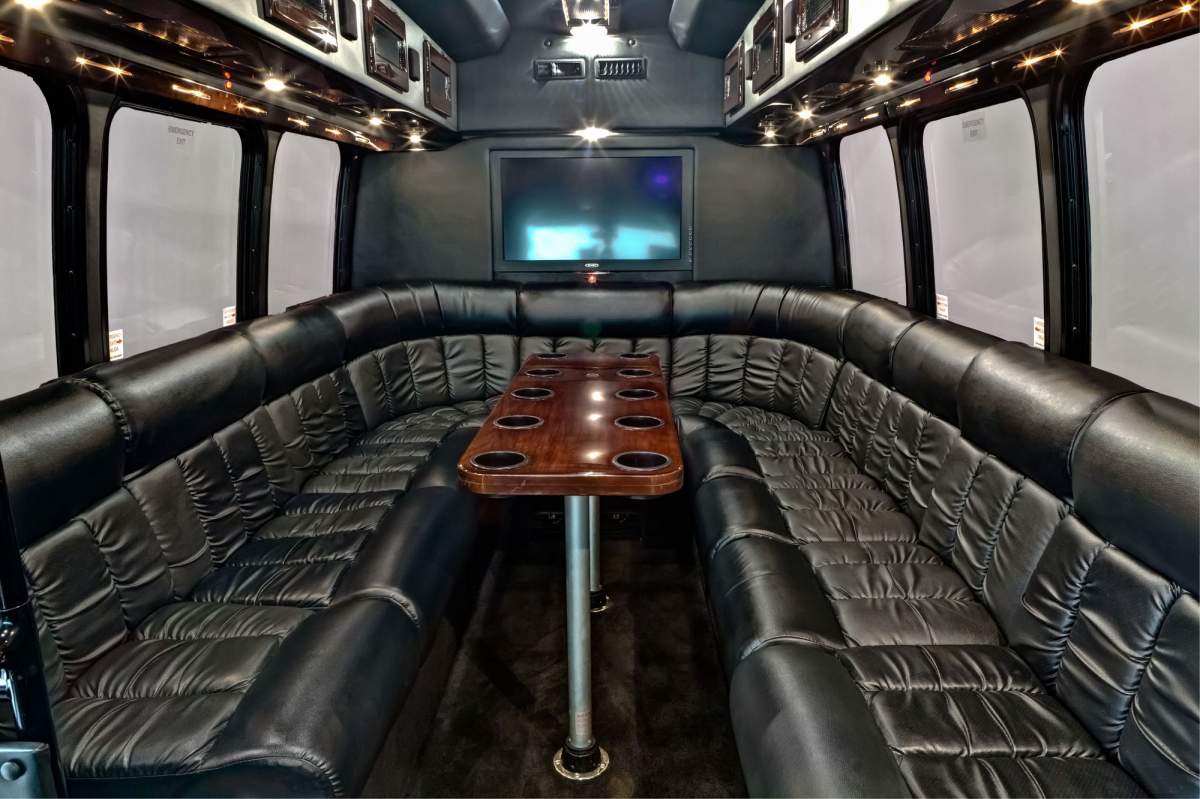This is an interior photograph of a luxurious party bus or limousine. The scene is dominated by a U-shaped arrangement of black leather seats, inviting guests to sit along the perimeter of the vehicle. Intricately positioned in the center of this U-formation is a dark red wooden table, supported by two silver poles, featuring 10 cup holders—five on each long side—perfect for holding drinks during lively gatherings. The floor of the vehicle is a plush-looking velvet black, adding to the opulent atmosphere.

On both the left and right sides of the bus, fogged windows with a gray filter prevent the outside view from intruding, enhancing the intimate, cozy feel. Above the seating area, the ceiling is dotted with various lighting fixtures, creating a bright and inviting ambiance. The back wall of the vehicle hosts a built-in TV, framed by intricate reddish-brown faux wood decorations, lending a touch of sophistication. Additionally, overhead consoles with black screens and more lighting can be seen on both sides, illuminating the space below in a soft, welcoming glow. The overall setup, with its combination of functional cup holders, ambient lighting, and luxurious seating, makes it clear that this is a space designed for enjoyment and socializing.